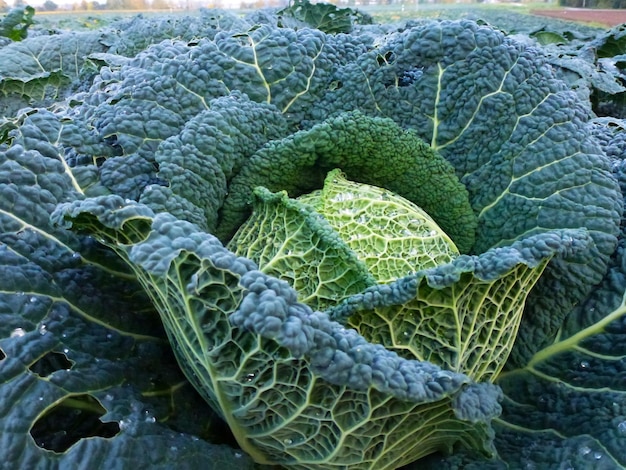This detailed, close-up photograph captures a large cabbage or a similar leafy green plant, taken outdoors during the daytime. The focus of the image is on the plant, which showcases a rich diversity of colors ranging from light greens at the center to darker greens and bluish hues towards the edges. The leaves of the plant fan out in a manner reminiscent of flower petals, providing a striking texture and intricate structure. Water droplets can be seen clinging to the textured surface of the leaves, enhancing their vibrant appearance.

The center of the plant features light green leaves, while the outer leaves vary from dark green to bluish green. The prominent veins are light green and visibly stand out, especially on the underside of the vertically oriented leaves closest to the camera. These veins create a intricate pattern that adds depth to the image. Some leaves show signs of being eaten, with bite marks possibly from insects.

In the background, there is a small town, adding a sense of scale and context to the photograph. The background also includes various trees and colors, framing the natural beauty of the plant life in the foreground. The scene appears to be set in a farm field, with a tree line visible on the left and an open field on the right, underlining the rural and serene setting of this image.